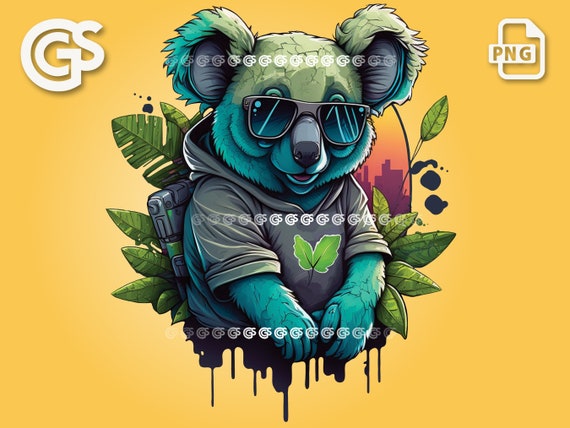This image showcases a cartoonish, teal-blue koala bear with a greenish top head and ears, positioned prominently at the center. The koala is adorned in a gray hoodie featuring a distinct graphic of two leaves on the front and dons a pair of stylish sunglasses. Surrounding the koala are numerous green tropical leaves set against a predominantly yellow background, with a cityscape and sunset subtly appearing on the right side. Adding to the scene is a dark liquid dripping from the koala's lower half. At the top left corner, there's a logo that reads "CS," while the top right corner is marked with "PNG" encased in a square. Throughout the image, the letters "GS" are subtly watermarked, enhancing its graphic charm.